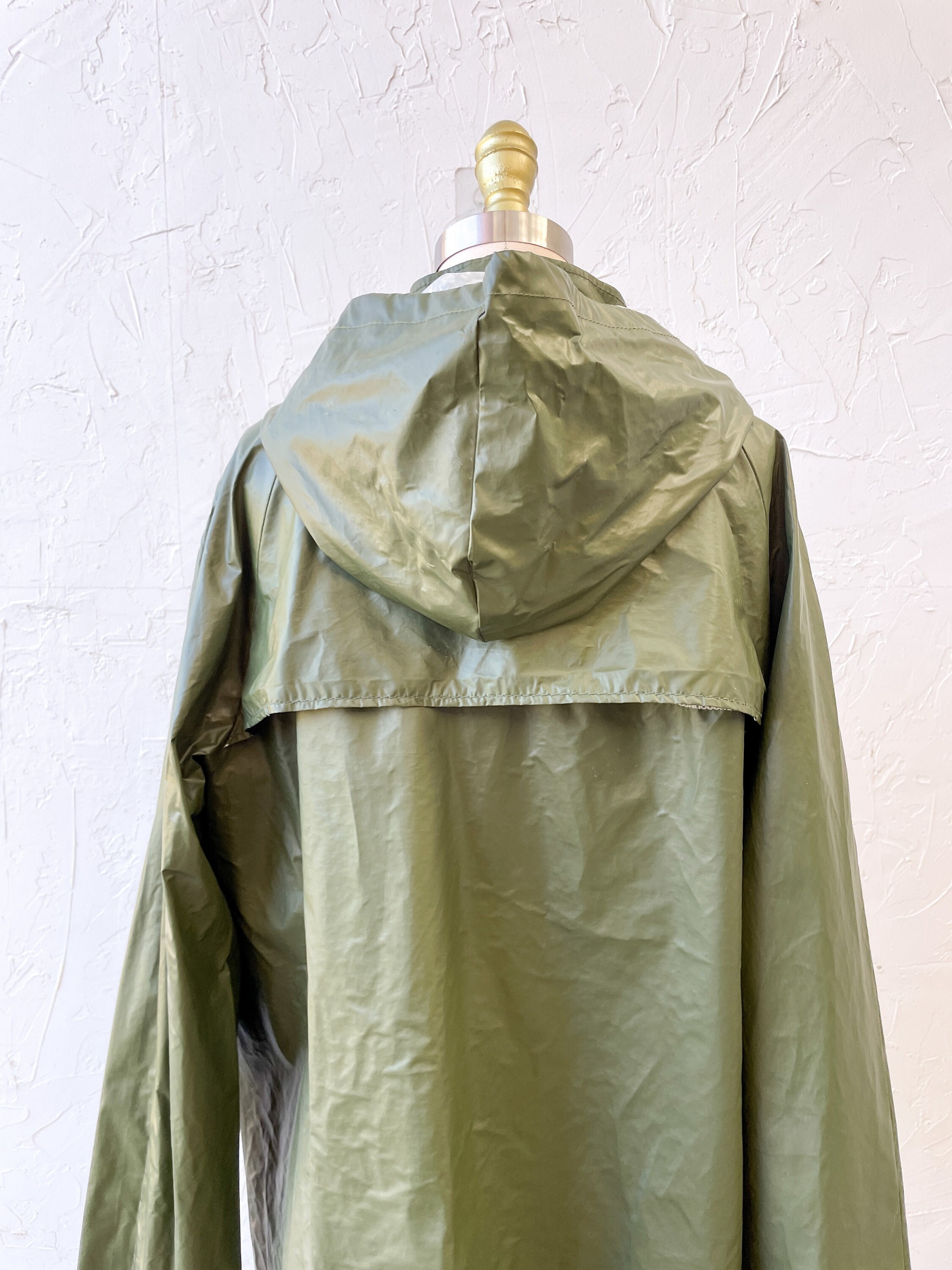The image features an olive green, hooded raincoat hanging on a rack against a white or beige wall with noticeable wear, including small cracks, scratches, and inconsistent paint layers. The coat is positioned on a rack or a mannequin torso, which is topped with a gold knob and encircled by a silver band. The raincoat is notably wrinkled, suggesting it has either been washed recently or not hung properly. The back of the coat is visible, showcasing a flap and a crease along the center, with particular folding on the upper left back. The coat appears to be designed for a taller individual, given its long sleeves, and reflects a yellowish light, further emphasizing its drab, olive grey hue.